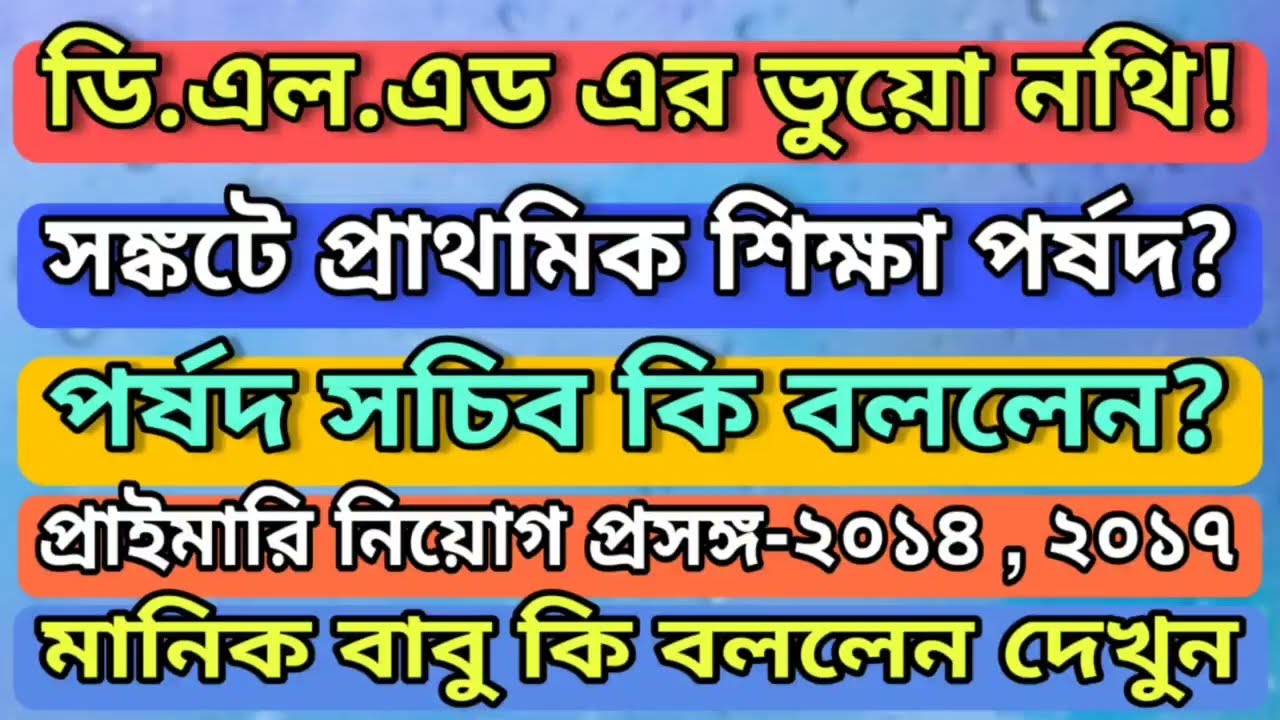The image showcases a simple yet vibrant graphical design featuring text in Hindi. It has a solid blue background accented with subtle, blurred water droplets near the top, adding a touch of texture. The design consists of five rows of multicolored rectangular text boxes with rounded corners, each casting a shadow onto the rectangles beneath them. 

From top to bottom, the rectangular backgrounds are red, dark blue, orange-yellow, light red, and light blue. Correspondingly, the text colors are yellow with a black outline, white with a black outline, blue-green with a black outline, white with a black outline, and yellow with a black outline. The text appears to be in Hindi, with punctuation marks at the end of some lines: the first row ends with an exclamation point, the second and third rows end with question marks, the fourth row ends with a comma, and the fifth row has no punctuation.